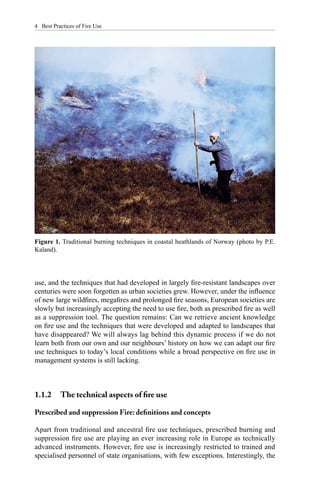The image depicts a slightly blurry article titled "Best Practices of" with the remaining title unclear. The article features a picture identified as Figure 1 and captioned "Traditional Clothing Techniques in Coastal Southlands of Norway" or possibly "Traditional Burning Technique." The photograph shows an elderly person, seemingly a man based on multiple accounts but potentially an older woman, dressed in a blue jacket or sweatshirt and black pants. The individual, slightly hunched, leans on a tall stick, perhaps around 7 feet in height, which might indicate frailty or a support tool for traversing rugged terrain. The person also wears a white scarf around their head. The scene is set amidst significant fog or possibly mist from the ocean, making the environment look murky, especially in the upper half of the image, while the bottom half reveals beat-up, brownish grass. The edge of the landscape suggests proximity to either a foggy coastal area or an incoming wave, contributing to the overall desolate and mysterious mood of the photograph. Text underneath mentions "photo by P.E." (last name unclear) and discusses the development and use of unspecified traditional techniques.